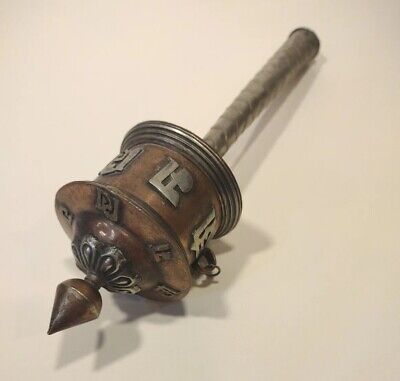The image depicts a metal dreidel, possibly made of bronze or copper with silver or pewter accents, resting on its side against a light cream background. The dreidel features a cylindrical body adorned with Hebrew letters and has additional Hebrew inscriptions underneath the cylinder. The handle, extending from the top right to the middle of the image, is a medium length, straight pole that widens at the top and narrows toward the dreidel. The handle appears to be crafted from woven fibers, although it is actually metal, and presents a silver or pewter finish. The dreidel has an ornate, cone-shaped floral finial at the bottom that serves as the spinning point. The top of the cylinder is crowned with ringed, molded decorations, adding to its intricate design, giving the dreidel a ceremonial and medieval appearance.